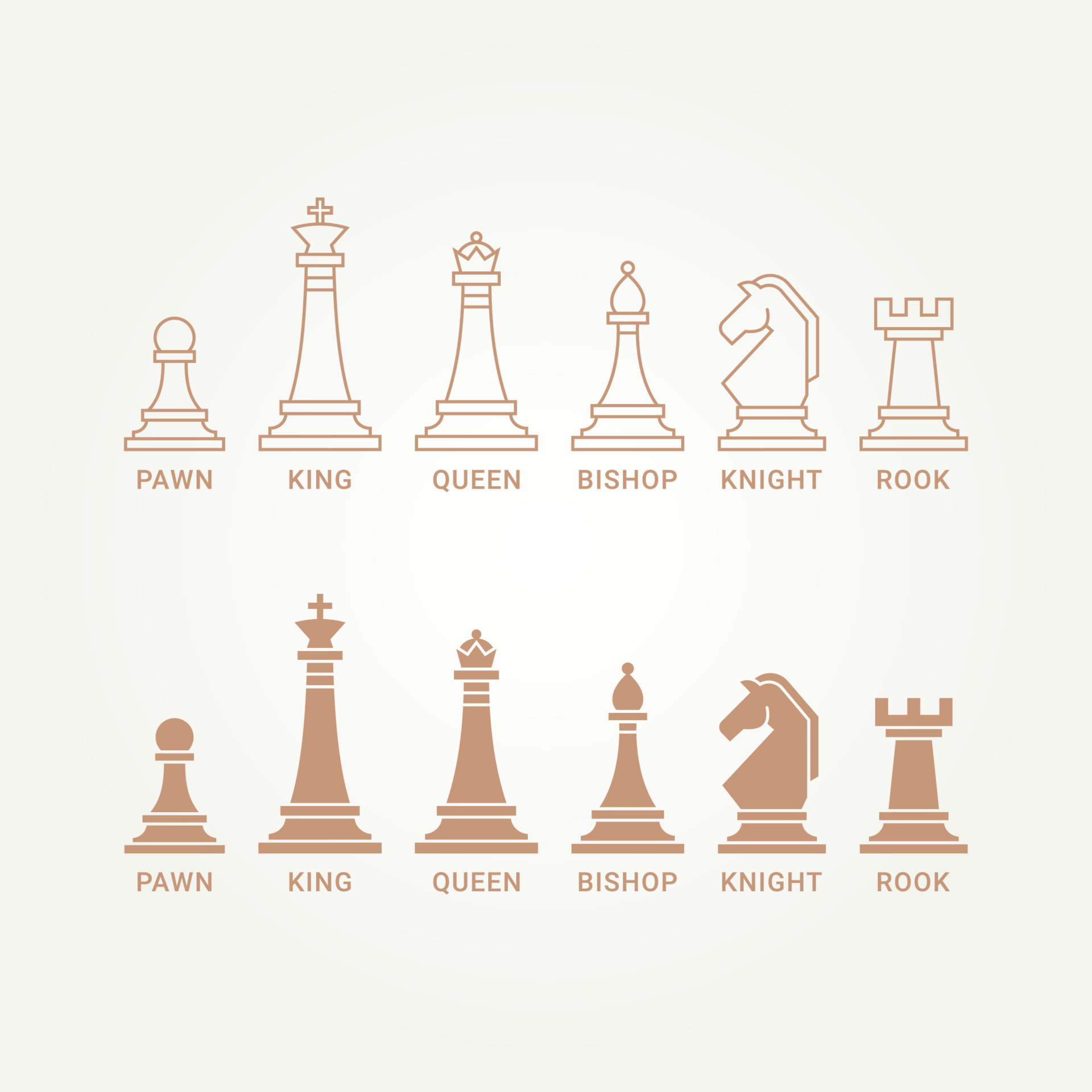This image is a detailed monotone illustration of chess pieces set against a white square background. The chess pieces are depicted in a light reddish-brown color. At the top, the illustration features the white pieces, which are simply outlined. These include the pawn, king, queen, bishop, knight, and rook, labeled in that order from left to right. Similarly, at the bottom, the illustration shows the black pieces, which are the same images but filled in with the reddish-brown color. They are also labeled from left to right as pawn, king, queen, bishop, knight, and rook. This comprehensive and clearly labeled infographic provides a clear representation of the different chess pieces used in the game.